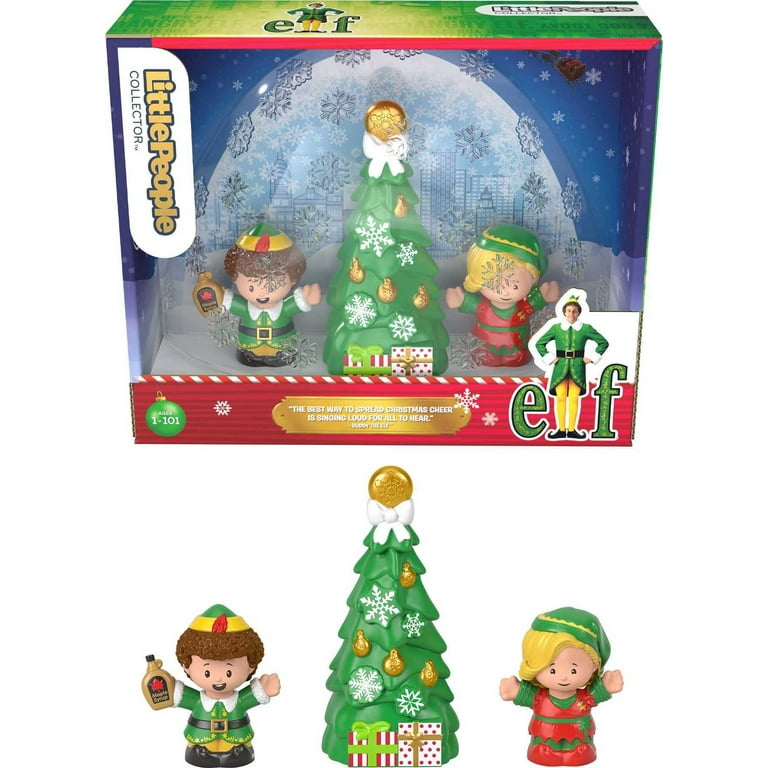The image depicts a color photograph of a gift set for the Christmas movie "Elf" starring Will Ferrell. The photograph, in portrait orientation, captures the packaged toy set prominently in the top half, encased in a green and red holiday-themed box. The front of the box is transparent, revealing the three toy figures inside. On the bottom right corner of the box's front, an image from the movie displays the "Elf" logo, where Will Ferrell's character stands as the "L" in "Elf." 

At the top left, the text "Little People Collector" is printed, and below the clear section, the phrase "The best way to spread Christmas cheer is singing loud for all to hear" is prominently featured. The three central components of the set consist of a Christmas tree adorned with white snowflakes and gold ornaments, topped with a circular globe, flanked by two elf figures. To the left is a blond-haired elf wearing a red outfit with a green hat, while the right side shows a darker-haired elf resembling Will Ferrell, dressed in a green and yellow outfit with a red-trimmed green and yellow helmet, holding what appears to be a condiment bottle.

Below the packaged set, the individual toy figures are displayed out of their wrapper against a white backdrop. The left figure is a little elf boy in green and yellow clothing, the middle is the decorated Christmas tree, and on the right is a young elf girl dressed in green and red attire. Both elves are depicted smiling with their arms raised.